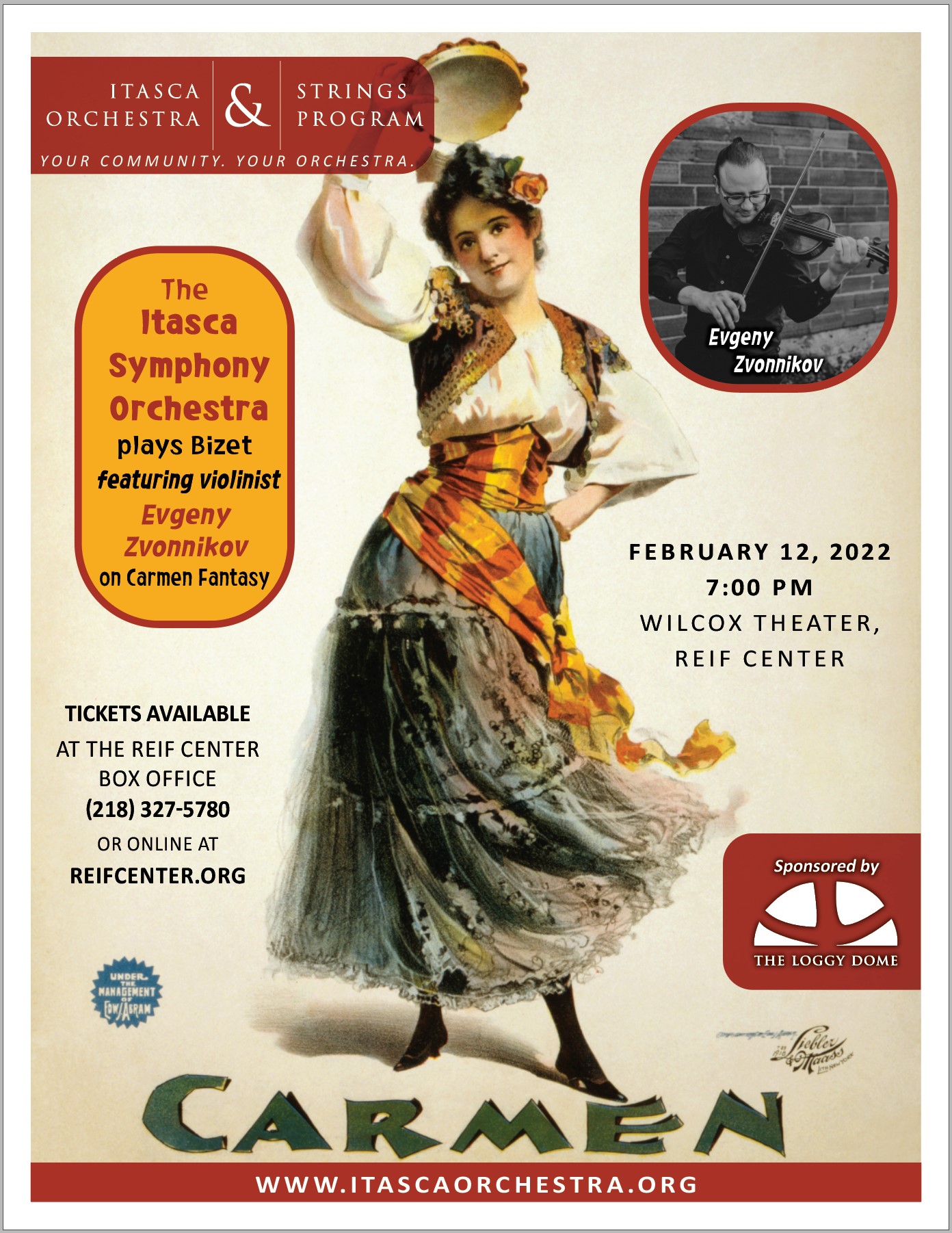The poster promotes the Itasca Symphony Orchestra's performance of Bizet's Carmen, featuring renowned violinist Evgeny Svonikov on Carmen Fantasy. At the top left corner, it states "Itasca Orchestra and Strings Program, Your Community, Your Orchestra." Featured prominently in the middle is an art depiction of a woman, "Carmen," adorned in a vibrant costume: a black dress with a yellow and red sash, a red vest, a white blouse, and a floral headpiece. The right corner of the poster showcases a photo of Evgeny Svonikov, highlighting his participation. The bottom of the page provides the website, www.itascaorchestra.org, and notes that the event is sponsored by the Loggie Dome. The details indicate the performance date as February 12, 2022, at the Wilcox Theater, with box office information available.